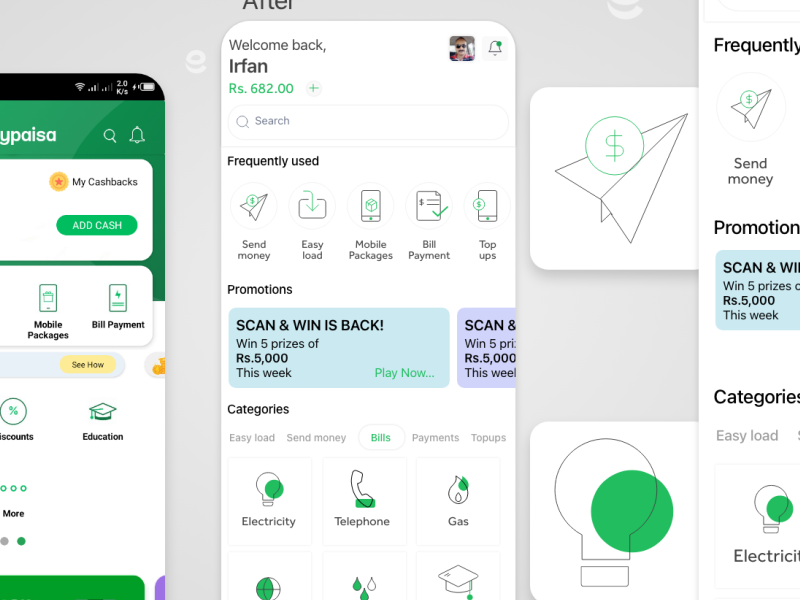This image is a composite of multiple smartphone screenshots displayed side by side.

On the left, there is a partial screenshot featuring a color scheme of green, white, yellow, and black. The visible text includes "My Cashbacks" and a green button labeled "Add Cash." There are also several icons: a green iPod icon for "Mobile Packages," another for "Bill Payment," an "Education" button, and a "Discounts" button.

The central screenshot welcomes a user named Irfan and includes a small picture of a man next to the greeting. Below this, there are options with corresponding icons: "Send Money," "Easy Load," "Mobile Packages," "Bill Payment," and "Top-Ups." There's also a promotional banner stating "Scan and Win is Back! Win five prizes of RS 5000 this week," ending with a "Play Now" button. Further down, there are categories listed: "Easy Load," "Send Money," "Bills," "Payments," and "Top-Ups." Following these categories are icons representing various utilities: a light bulb for "Electricity," a telephone handset for "Telephone," and a drop for "Gas." Additional icons are present but not legible.

On the right side, there is a large white light bulb icon, representing "Electricity," depicted within a green circle. Underneath, sections labeled "Promotions" and "Categories" are visible.